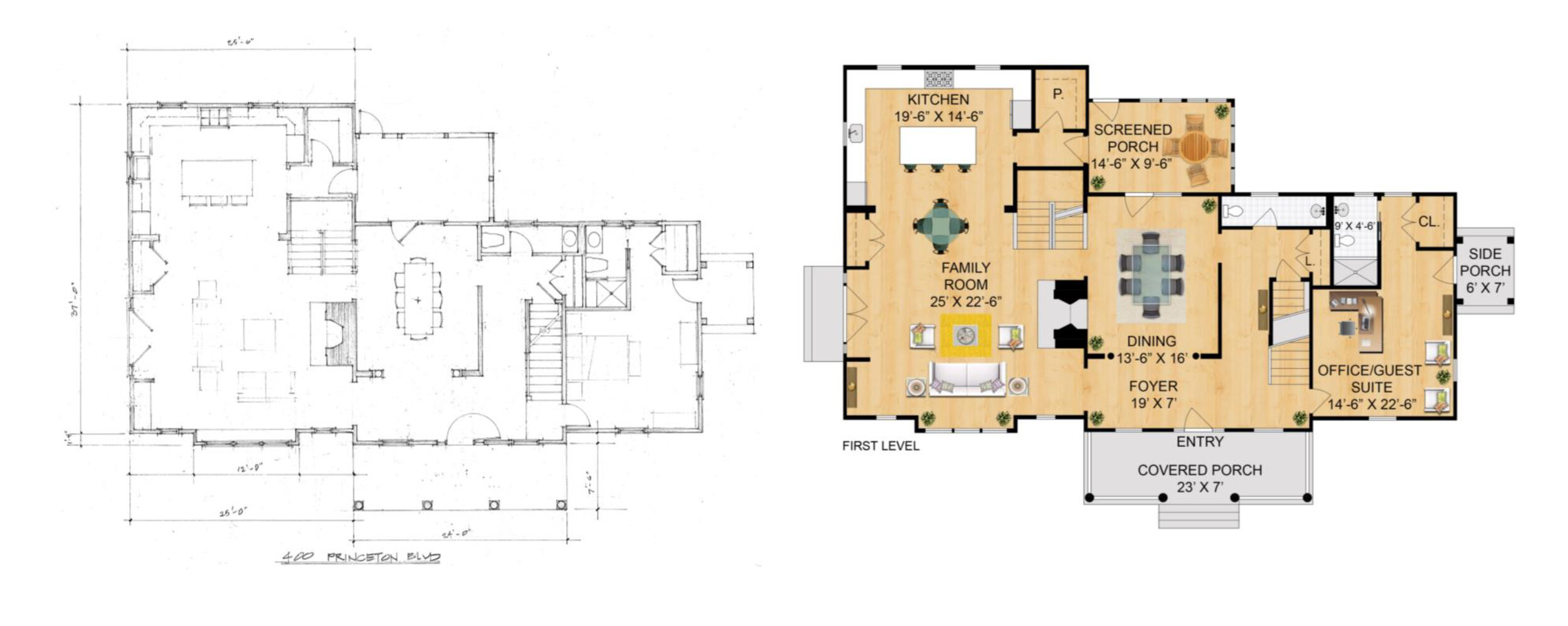The image features two distinct architectural drawings of a house layout. On the left, there is a classic black and white blueprint with a white background and black cutout lines, showcasing a simple yet precise drawing of the house's structure. Exterior and interior measurements also appear around and within this layout. Conversely, the right side displays a more vibrant, color-enhanced version of the same layout, resembling a computerized drawing. This version fills in details such as wood-colored floors, multicolored furniture (including yellow, green, and orange), and additional labels marking various rooms and porches in black lettering. Detailed room dimensions are provided: the kitchen measures 19 feet 6 inches by 14 feet 6 inches, the screen porch is 14 feet 6 inches by 9 feet 6 inches, the family room spans 25 feet by 22 feet, the dining room is 13 feet by 16 feet, the foyer is 19 feet by 7 feet, the office guest suite is 14 feet by 22 feet, and the side porch is 6 feet by 7 feet. Labels also indicate other areas like a covered porch, emphasizing it is all on the first level of the building with the address 400 Princeton Boulevard.